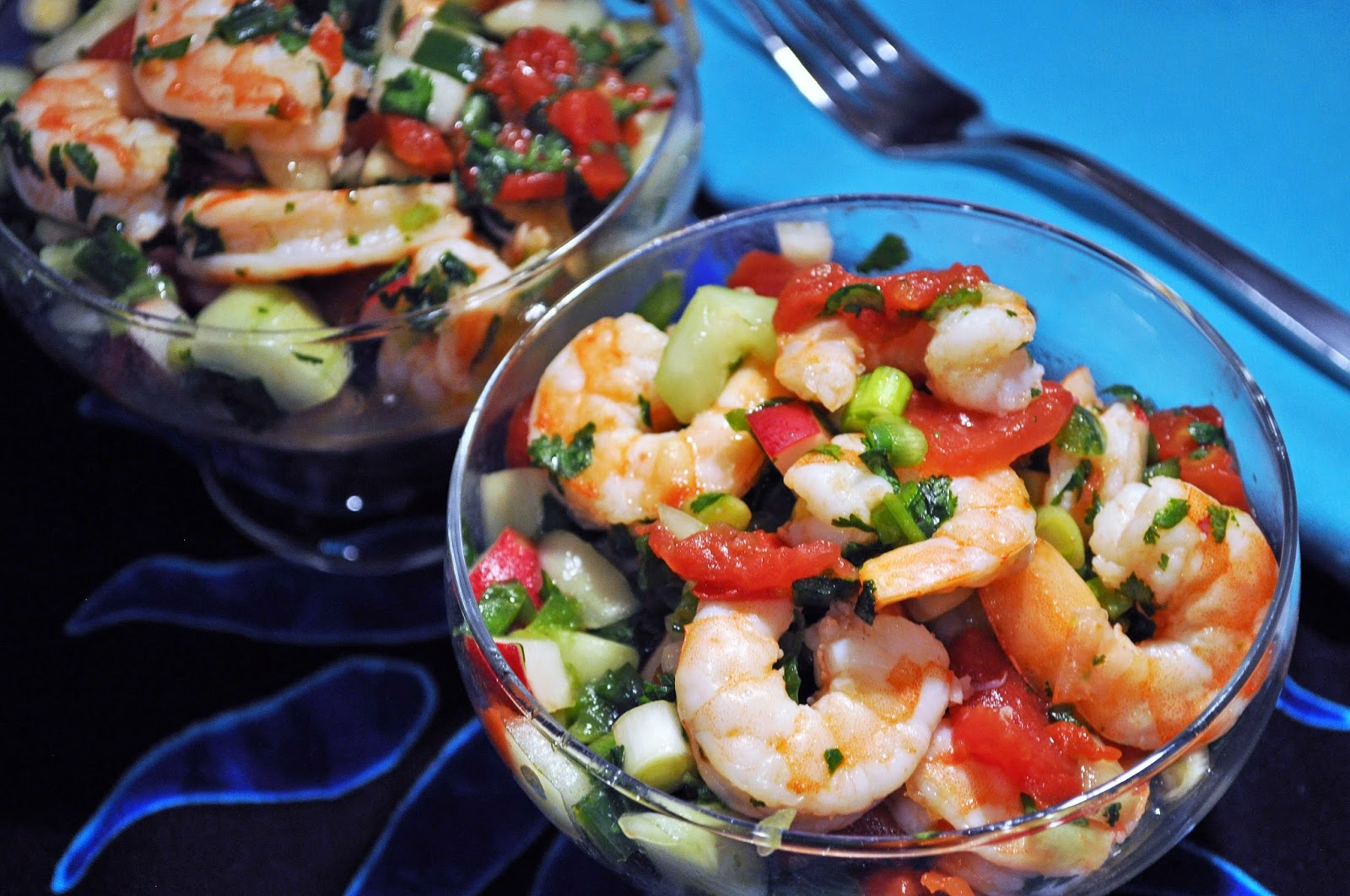The image depicts a beautifully presented shrimp salad served in two transparent glass bowls resembling shrimp cocktail glasses. The vibrant salad is a colorful mixture of shrimp, tomatoes, corn, green onions, peppers, and leafy greens, garnished generously to enhance its appeal. Behind the bowls, a silver fork rests on a sky blue napkin, providing a pop of color against the dark tablecloth adorned with dark blue, flame-like floral patterns. The bowl on the right is in focus, serving as the main subject of the photograph. The setting, possibly in a restaurant, showcases a meticulous arrangement that highlights the freshness and seasoning of the salad, making it an enticing visual feast.